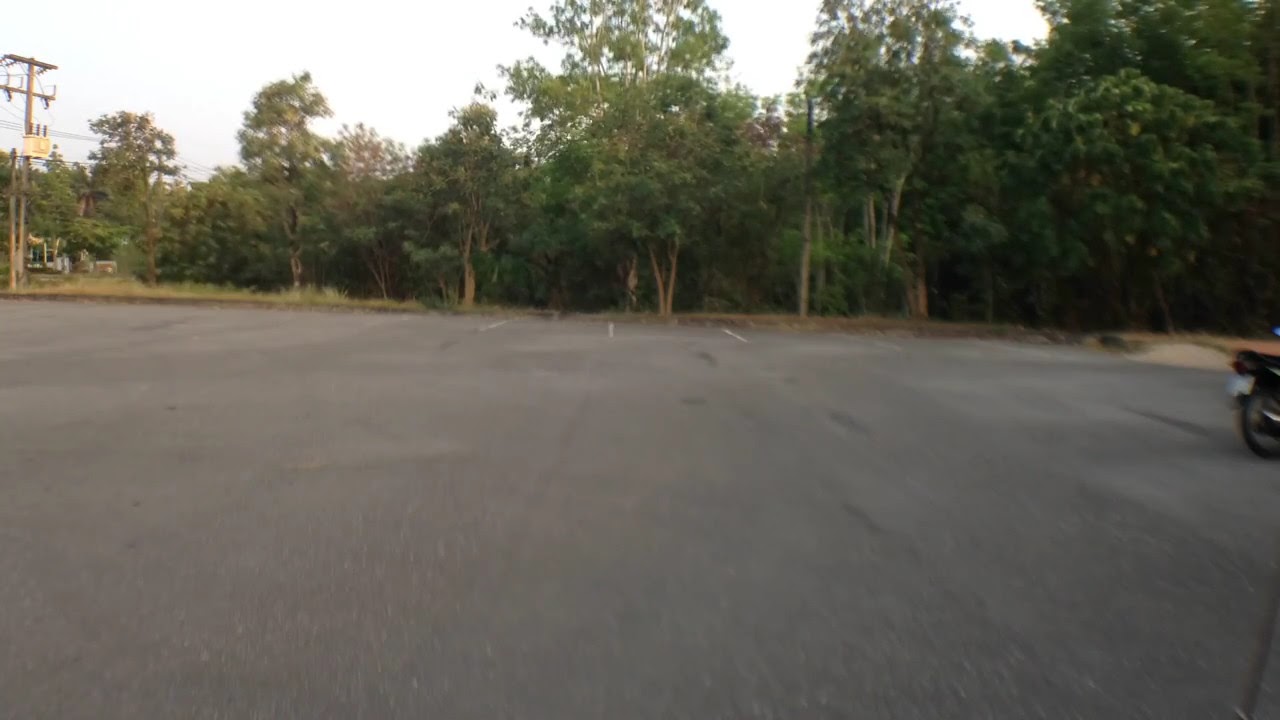This photograph captures a quiet, empty asphalt parking lot on a cloudy day, giving the scene a dark and dreary feel. The lot is marked with white lines designating parking spaces, and the view is primarily dominated by the gray concrete pavement. A single motorbike or moped, with only its back wheel, seat, and license plate visible, is parked on the right side of the image. Lining the back of the lot is a row of green trees that add a touch of nature to the otherwise nondescript scene. On the left side of the photograph, utility poles and power lines are visible, stretching horizontally across the image. In the distance, there are small buildings partially obscured by the trees. The sky overhead is overcast, contributing to the somber and subdued ambiance of the setting.